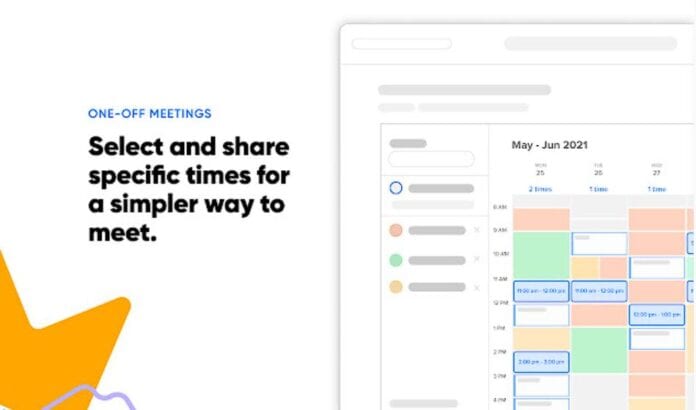The image features a white background. On the left side, the title "One-off Meetings" is prominently displayed in blue text. Below this, in black text, the caption reads: "Select and share specific times for a simpler way to meet." In the bottom left corner, there's a partially opened yellow file folder, which is bifurcated and contains a purple squiggly line. 

On the right side of the image, there is a calendar for May and June 2021. The calendar's time slots range from 8 a.m. to 4 p.m. down the left side. The specific date shown is Monday, June 25th, but adjacent dates—June 25th, 26th, and 27th—are also visible moving horizontally across the calendar. The calendar is filled with various blocks of color: pink, green, and blue. The blue blocks contain text that is mostly unreadable and appears as gray lines or squiggles, likely due to low resolution or intentional design for a quick visual glance rather than detailed reading. The clearly readable elements include the months "May June 2021" and the time slots. The overall design seems intended to provide a general visual representation rather than detailed information.